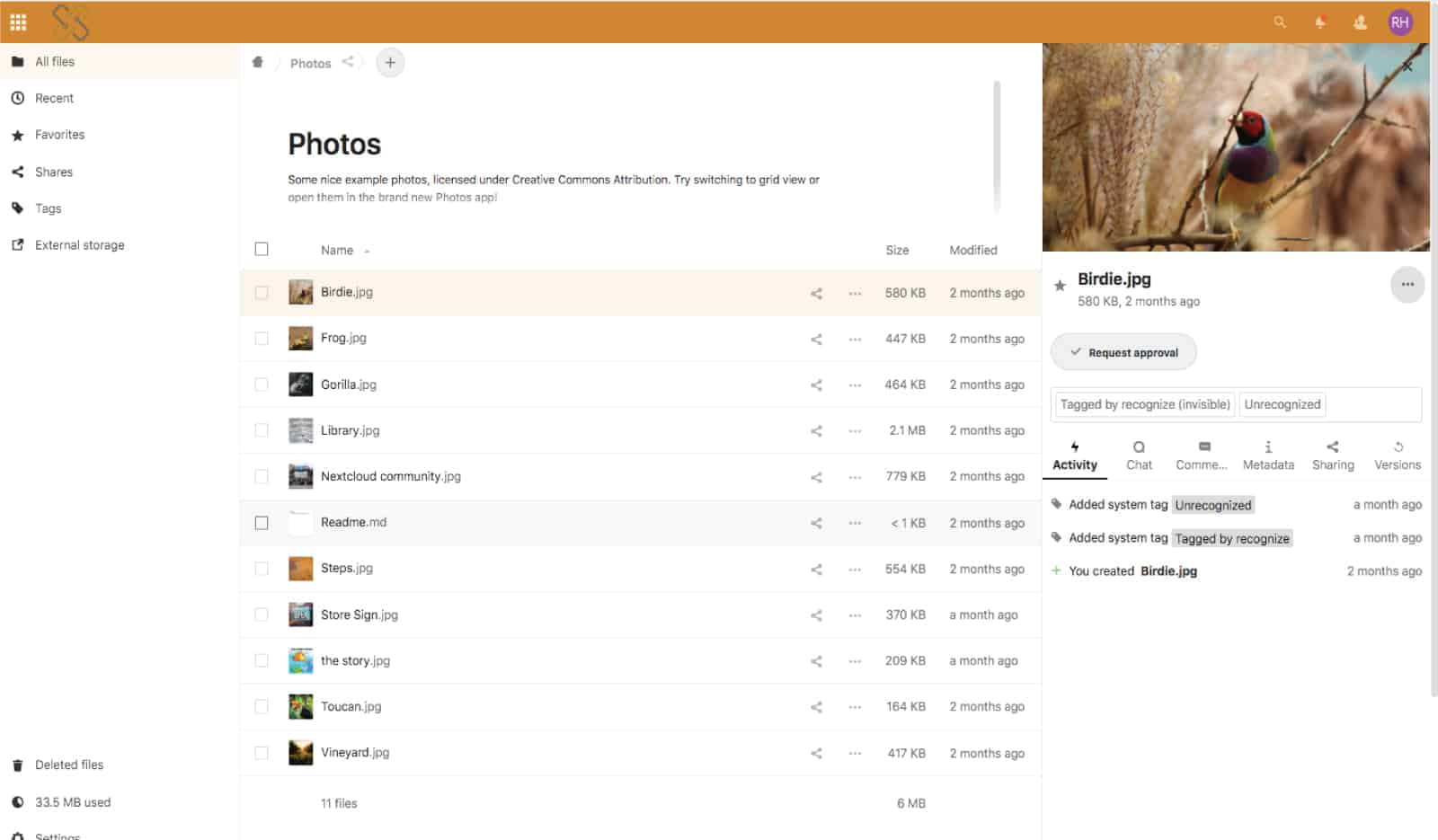A user is viewing photos on a desktop screen that is split into multiple sections for navigation and detailed information. To the left of the screen is a navigation panel featuring categories such as "All Files," "Recent," "Favorites," "Share," "Tags," and "External Storage." Currently, the "All Files" category is selected, indicated by its highlighted appearance.

The central portion of the screen, which occupies the majority of the view, displays the "Photos" section. At the top of this section are icons for sharing and adding files. The header in bold black text reads "Photos," with a subheader in smaller text stating, "Some nice example photos, licensed under the Creative Commons Attribution. Try switching to grid view or open them."

Below this, the content area lists various image files, each with details organized under columns labeled "Name," "Size," and "Modified." The files include "birdie.jpg," "frog.jpg," "gorilla.jpg," "library.jpg," and "nextcloud.jpg," among others, totaling approximately 12 files. Each file entry includes a small thumbnail preview, file size, and last modified date. For example, "birdie.jpg" has a size of 580 kilobytes and was modified two months ago.

To the top right of the screen, a larger preview of the selected image, in this case, "birdie.jpg," is displayed. This section also shows options for requesting approval, activity information like when the file was added, and its recognition status.

At the bottom of the left navigation panel, beneath the "External Storage" section, there is a hidden column revealing additional options such as "Delete File" mode and storage usage, which indicates 33.5 megabytes used. The "Settings" option is partially cut off at the very bottom of the panel.